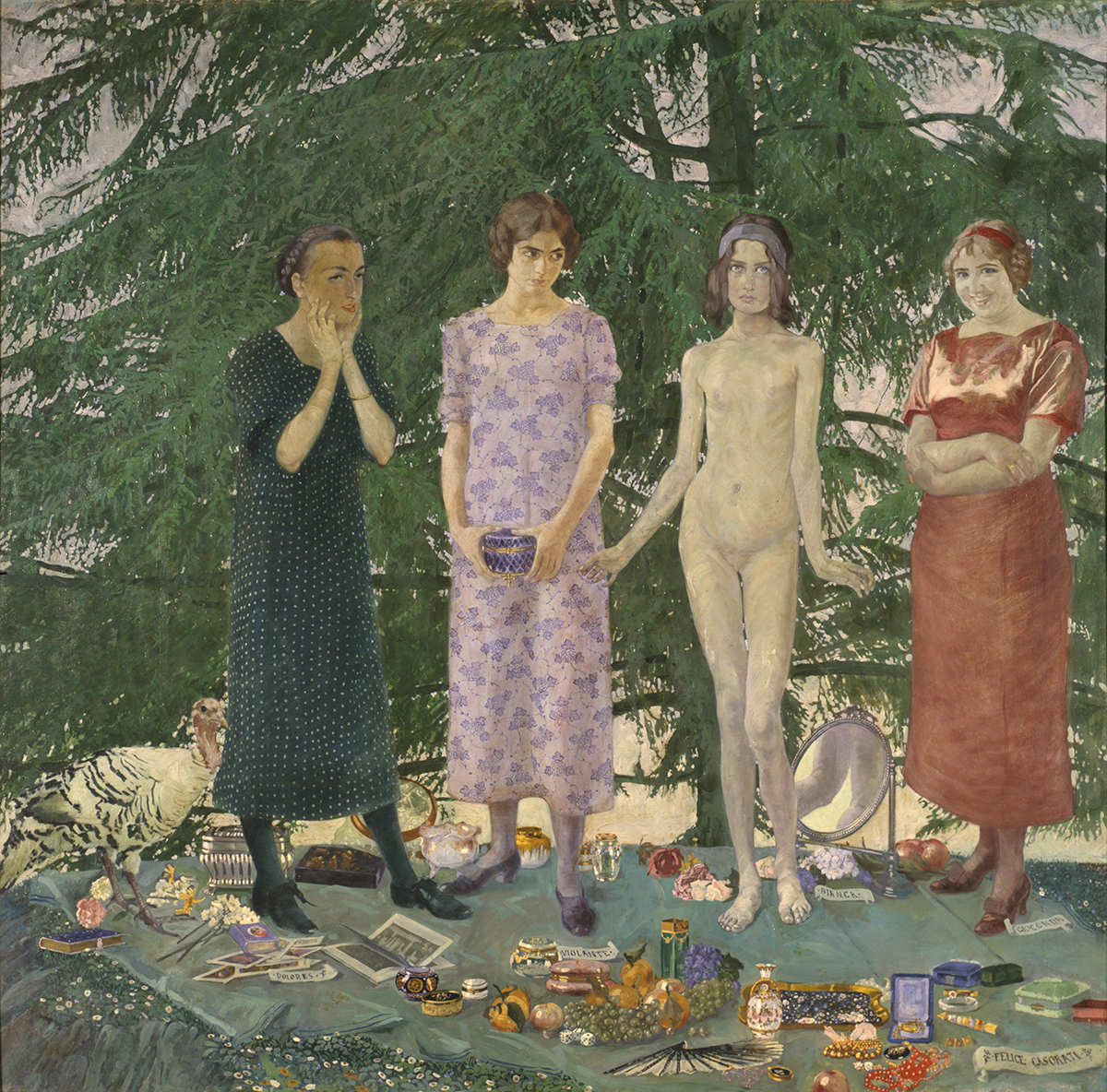The painting depicts four women standing on scattered objects beneath a large tree that spans the background. The leftmost woman wears a dark green dress with polka dots and has her hands on her face, her braided hair pulled back. Next to her, a woman in a light purple, floral-patterned dress holds an object at her hips, seemingly looking askance. The third woman stands naked, adorned only with a purple headband in her long brown hair, her hands resting by her hips. The rightmost woman, wearing an orange-red dress, smiles at the viewer. Underfoot, an assortment of items is strewn across the ground, including a hand fan, fruits, books, jewelry, makeup bottles, jars, tins, and cards. Near the green-dressed woman, a white bird with dark green lines and a brown head, resembling a hen, stands among the clutter. The painting is nearly square in shape.